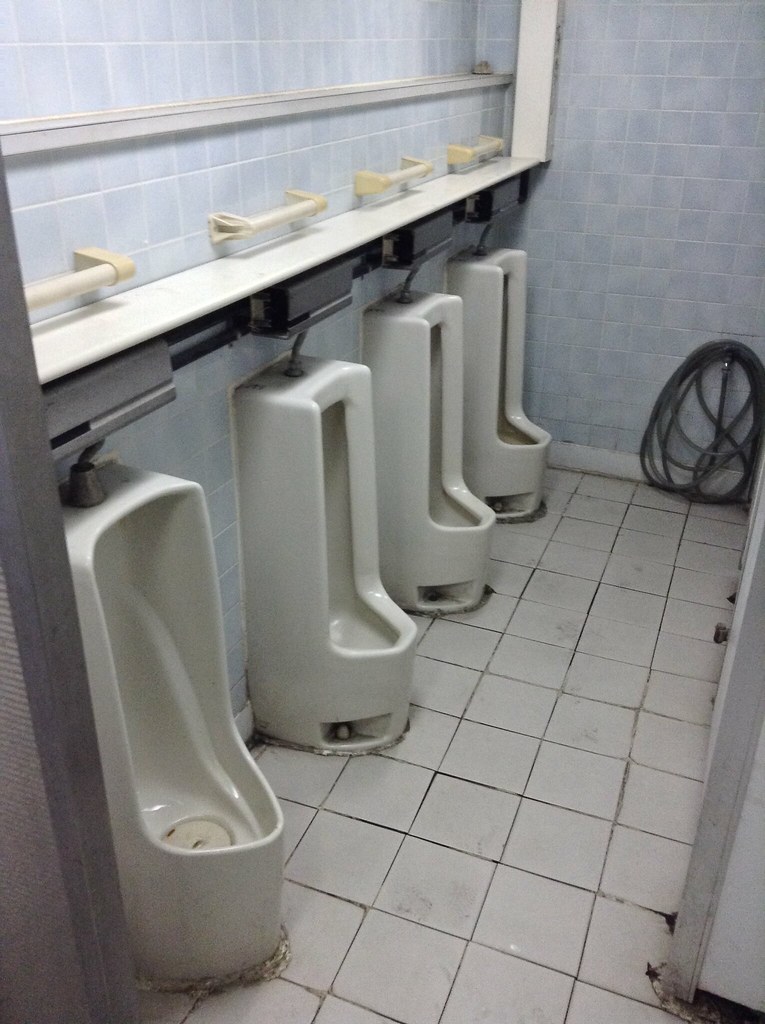The photo showcases a public men's bathroom with four white, ceramic urinals aligned in a row. Each urinal is deeply set and positioned above a dirty, tiled floor displaying a patchwork of cream, blue, and white tiles, interspersed with dark grout lines. The floor appears to have rust marks, possibly from a heater on the right side. Broken tiles are noticeable in spots, adding to the overall dilapidated look. Blue tiles cover the walls adjacent to the urinals, keeping with the bathroom's color scheme. In front of each urinal, there are mysterious white handles whose purpose remains unclear. Additionally, a black cord is seen lying in the corner of the room, further contributing to the room's cluttered and neglected appearance. The image captures the bathroom in a portrait orientation, highlighting both the vertical layout and the conspicuous state of uncleanliness.